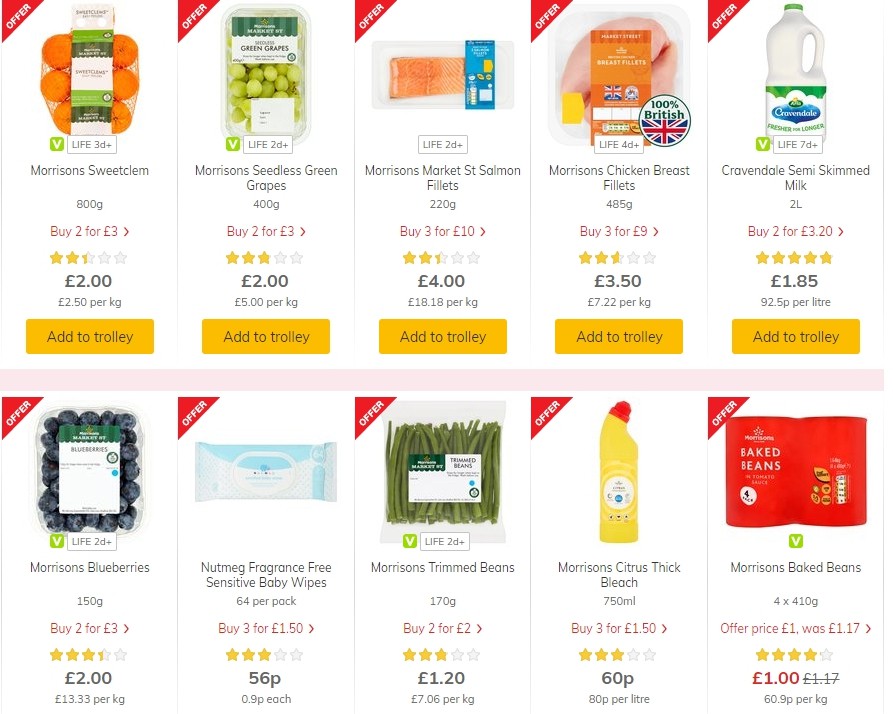This screenshot displays a grid of ten different food items arranged in two rows of five. Each item features a red triangle-shaped symbol in the top-left corner that says "OFFER" in white letters. At the bottom of each item, there is an orange rectangle with the text "ADD TO TROLLEY."

- The first item in the top-left corner is a bag of oranges labeled "MORRISON'S SWEET CLEM 800 grams." The offer details state "Buy two for three pounds." This item has a rating of two and a half stars out of five, priced at two pounds, equating to 2.5 pounds per kilogram.
  
- The second item to the right is a plastic container of green grapes labeled "MORRISON'S SEEDLESS GREEN GRAPES 400 grams." This product also has an offer of "Buy two for three pounds," rated three out of five stars, with a price of two pounds, translating to five pounds per kilogram.

- The third item in the same row shows raw salmon, but the details continue beyond this snippet.

Each item in the grid follows a similar structure, prominently displaying both discounts and ratings to inform shoppers of their choices.